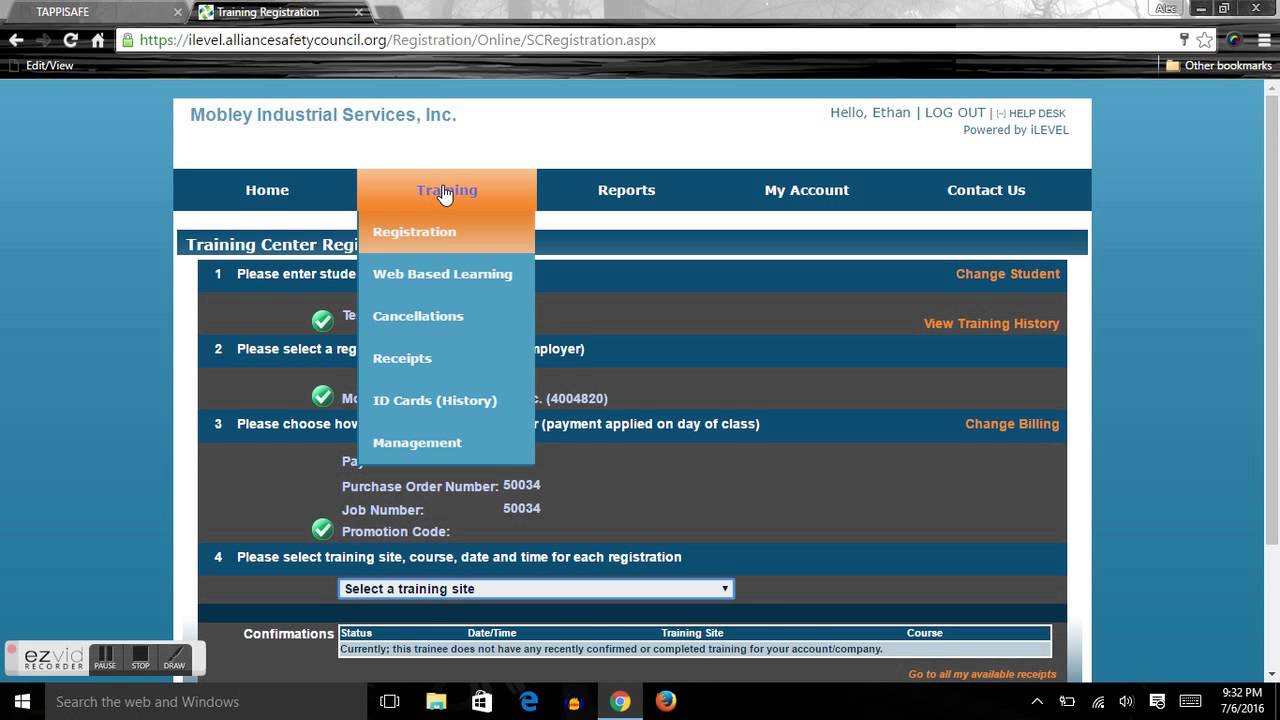This is a detailed screenshot of the Mobley Industrial Services Incorporated website interface. The screenshot features a clean white border that frames the top, left, and right sides of the page, while the background beyond these borders is a cohesive blue color. Across the top of this interface, the text "Mobley Industrial Services Incorporated" is prominently displayed. In the upper right-hand corner, there are several navigational options including "Hello Ethan," a link to "Log Out," access to the "Help Desk," and a note indicating the website is "Powered by iLevel."

Directly beneath this header, there is a horizontal menu bar offering navigation tabs such as "Home," "Training," "Reports," "My Account," and "Contact Us." The "Training" tab is currently selected, revealing a comprehensive drop-down menu. The options within this menu include "Registration," "Web-Based Learning," "Cancellations," "Receipts," "ID Cards," "History," and "Management."

Furthermore, located in the bottom left corner of the page is a button labeled "Easy Vid Recorder." This button provides additional functionalities including "Pause," "Stop," and "Draw," facilitating easy video recording and annotation for the user. The overall layout is user-friendly, with intuitive navigation and clearly defined sections for efficient user interaction.